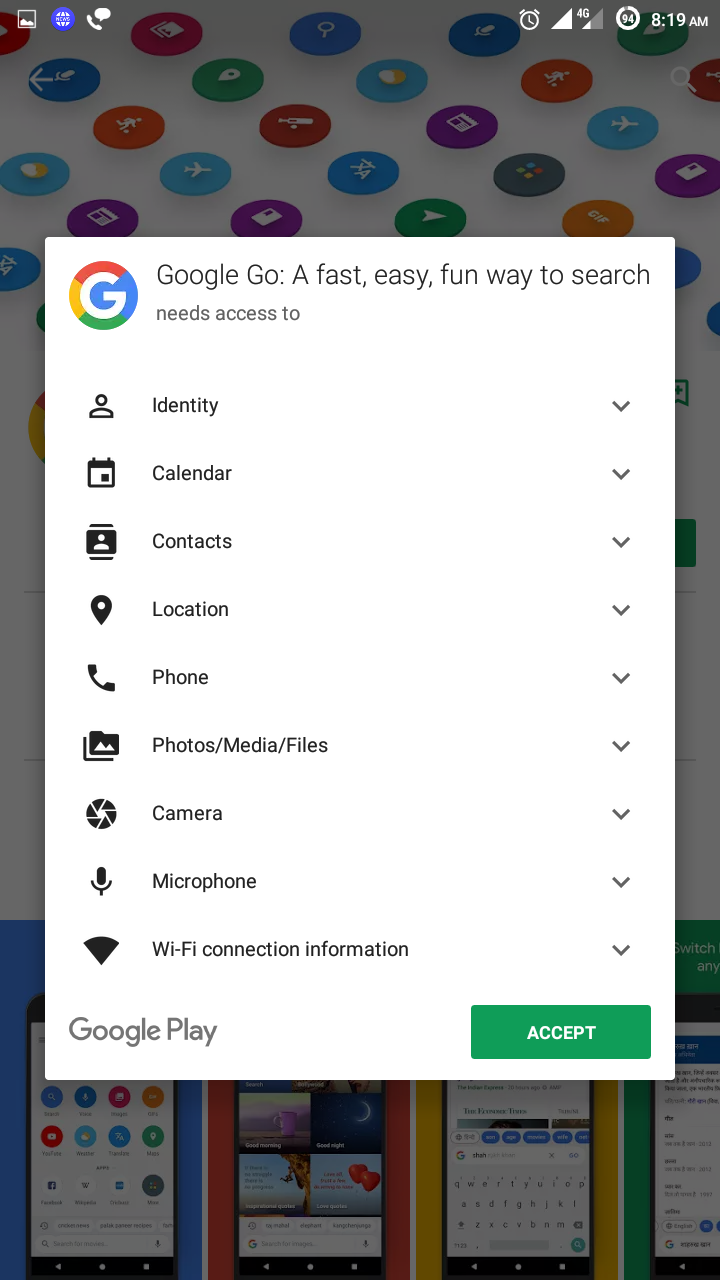The image is a screenshot taken from a smartphone. In the upper right-hand corner, the time is displayed as 8:19 AM in white font. The battery icon shows a 94% charge, and the device is connected to a 4G wireless network. The background of the screenshot is slightly grayed out, drawing attention to a central rectangular shape that is almost a square, in an off-white color.

At the very top of this central shape, the Google logo is prominently visible, comprising a white "G" encircled by segments in blue, green, yellow, and red. To the right of the logo, in gray font, the text reads, "Google Go, a fast, easy, fun way to search." Below this header, it states that the app "needs access to" a list of required permissions.

The comprehensive list of permissions includes:
- Identity
- Calendar
- Contacts
- Location
- Phone
- Photos/Media/Files
- Camera
- Microphone
- Wi-Fi connection information

Toward the lower right-hand corner of this off-white square, there's a green rectangle with white font that says "Accept."